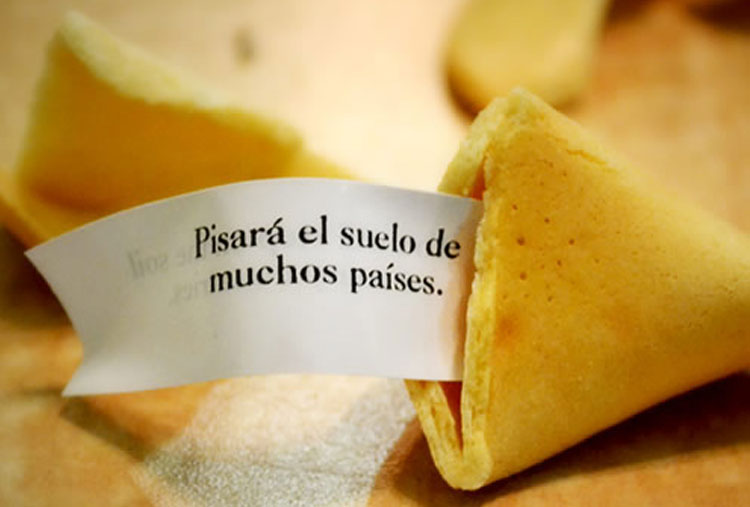The image is a close-up of a broken-open fortune cookie, with the visible half positioned prominently in the right-hand side of the frame forming a triangle shape. The cookie is light brown, and a crisp, white fortune extends from its center. Inscribed in black, capital letters, the fortune reads: "PASARÁ EL SUELO DE MUCHOS PAÍSES." The background features blurred, tan colors that may suggest other fortune cookies or a patterned cloth beneath the primary subject, though specific details are indistinct due to the tight focus on the cookie. The bottom portion of the image touches the edge of the frame, emphasizing the broken cookie and its message.